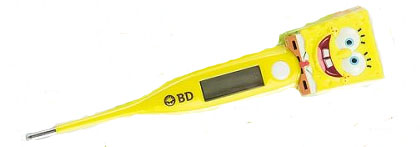The image depicts a children's thermometer featuring a Spongebob Squarepants theme, set against a plain, white background with no other elements. The thermometer has a design typical of oral thermometers, with a slender neck that culminates in a silver tip meant to be placed under the tongue. The body of the thermometer transitions from a narrow neck to a wider handle. 

The handle begins with the letters "BD" printed in black on a yellow background, followed by a gray digital readout screen, which is currently blank. There is a white button below the screen used to activate the thermometer. The design transitions into a detailed representation of Spongebob Squarepants, starting with his iconic brown shorts, white shirt, and red tie. 

The upper portion portrays Spongebob's yellow, sponge-like body with a big smile, showing his buck teeth and pink tongue. His large eyes, consisting of an outer white part and an inner blue section, are adorned with three eyelashes each. This lively depiction of Spongebob captures his cheerful and familiar appearance.